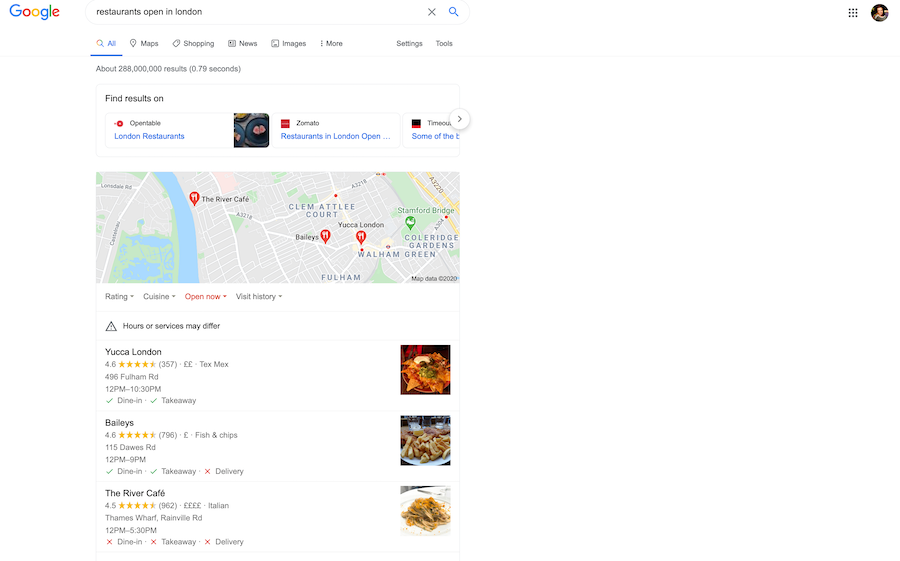The image appears to be a screenshot taken from a device, either a phone or a computer, showing a Google search results page. In the top left corner, the word "Google" is visible. Next to it, there is a search bar with the query "restaurants open in London" typed in. Below the search bar, a navigation bar presents options: "All," "Maps," "Shopping," "News," "Images," "More," "Settings," and "Tools," with the "All" option underlined in blue indicating it is the current selection.

Further down, the search results indicate there are approximately 288 million results found in about 0.78 seconds. The phrase "Find result on" is followed by "operation," then "London restaurants." 

A rectangular map is displayed prominently with three pinned locations highlighting specific restaurants in London that are currently open. Beneath the map, detailed information about the three restaurants is provided:

1. **Yucca London**: Rated at 4.8 stars, this restaurant offers Tex-Mex cuisine and serves dine-in and take-out options from 12 PM to 10:30 PM.
2. **Bailey's**: Known for its fish and chips, Bailey's has a rating of 4.6 stars and operates from 12 PM to 9 PM.
3. **The River Cafe**: Specializing in Italian food, this restaurant holds a 4.5-star rating. 

The information is presented in an organized manner, providing a quick yet comprehensive overview of dining options available in London.